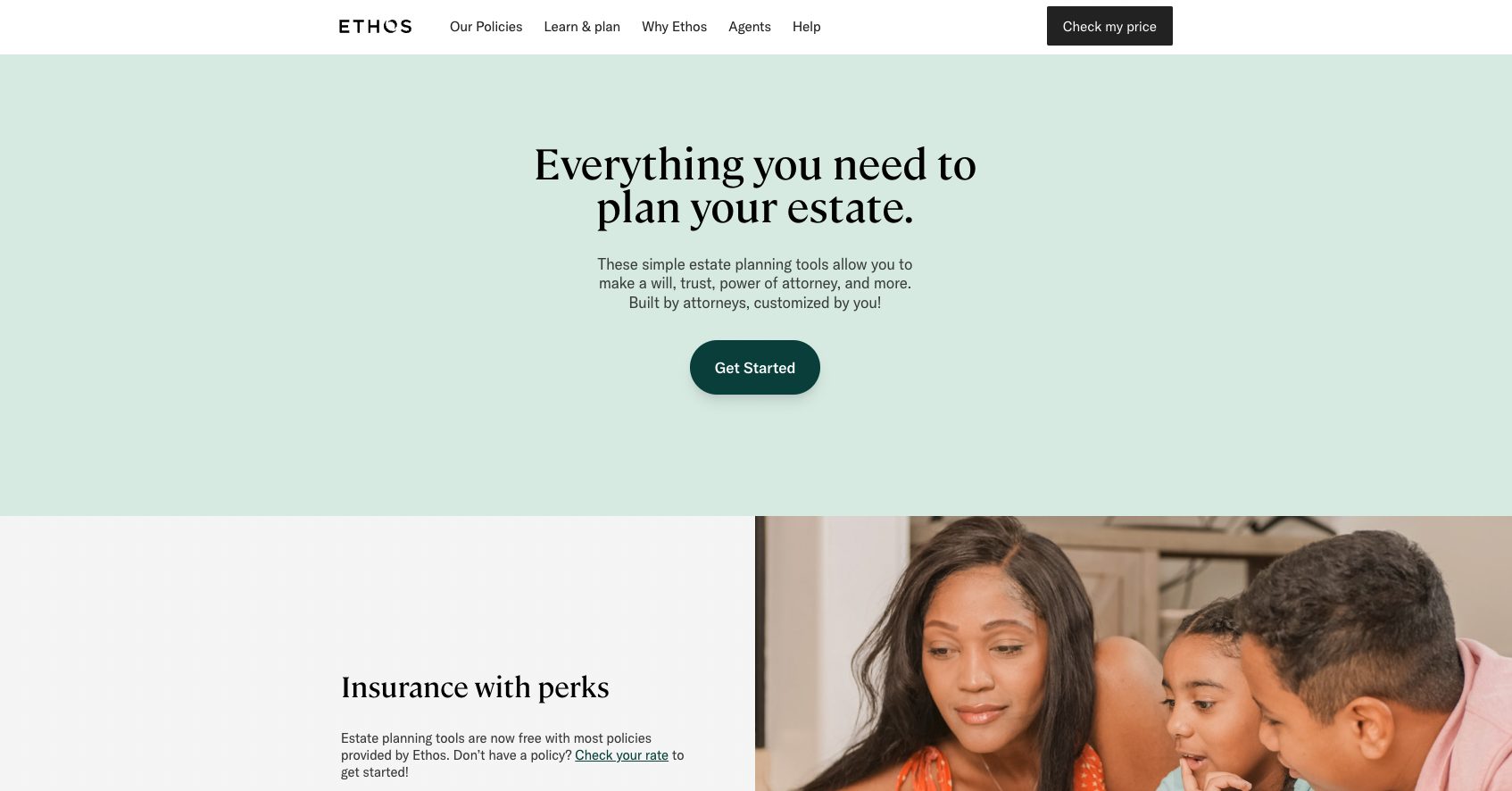Caption: The web page for Ethos boasts a user-friendly interface with clearly marked tabs at the top: Our Policies, Learn and Play, Why Ethos, Agents, and Help. To the far right, there is a prominent black button labeled 'Check My Price.' Below this navigation bar is a light pastel green section, featuring bold black text that reads, "Everything you need to plan your estate." This section emphasizes the simplicity and comprehensiveness of Ethos's estate planning tools, which include options to create a will, trust, power of attorney, and more. These tools are expertly crafted by attorneys but customizable to fit your unique needs. A prominent green 'Get Started' button invites users to begin.

At the bottom of the page, a gray section with black text announces, "Insurance with Perks: Estate planning tools are now free with most policies provided by Ethos." For those without a policy, a convenient link is available to check their rate and get started.

The page also features an engaging image of a mother, likely of African American descent, and her two children, who appear to be biracial. They are gazing intently at something, suggesting they are at home. The children, a girl and a boy, seem to be around seven and nine years old, respectively. The overall theme of the web page highlights Ethos's commitment to providing comprehensive and accessible estate planning solutions for families.